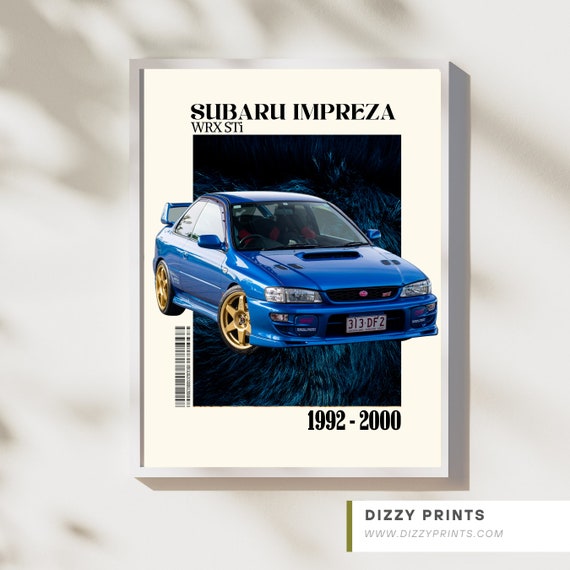This image is a detailed poster for a Subaru Impreza WRX STI from 1992 to 2000. The top of the poster prominently displays the title "Subaru Impreza WRX STI" in black letters against a black background with bluish tones. Superimposed over this background is a picture of a bright blue, two-door Subaru Impreza WRX STI with gold rims and a distinctive spoiler on the back. The visible license plate reads "313-DF2." On the left-hand side of the poster, there is a barcode located underneath the car image. At the very bottom of the poster, the years "1992-2000" are printed in black. Additionally, the lower right-hand corner features the text "Dizzy Prints" with the website "www.dizzyprints.com."